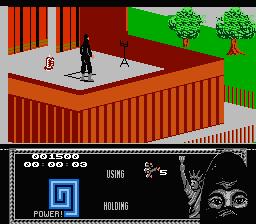The image depicts an 8-bit pixelated video game scene featuring a character in a black ninja outfit with light-colored boots and a dark head covering, evoking the style of early Nintendo and Sega games. The backdrop includes green grass and trees with large green leaves, bordered by a brown and orange picket fence surrounding a brown wooden deck with a white carpet in the center. The ninja character stands on the deck, seemingly focusing on a tripod-like object. In the foreground, there’s a long black box containing pixelated elements, including the outlined and gray-colored Statue of Liberty, and white text and numbers such as "001500," "using and holding," and "POWER" displayed in a blue curly font. An image of a masked face, with only the eyes and eyebrows visible, is also part of the interface, alongside a depiction of five little men, suggesting lives or characters available in the game. The scene incorporates elements of a maze in blue and dark blue, further enhancing the game's nostalgic, early-video-game ambiance.